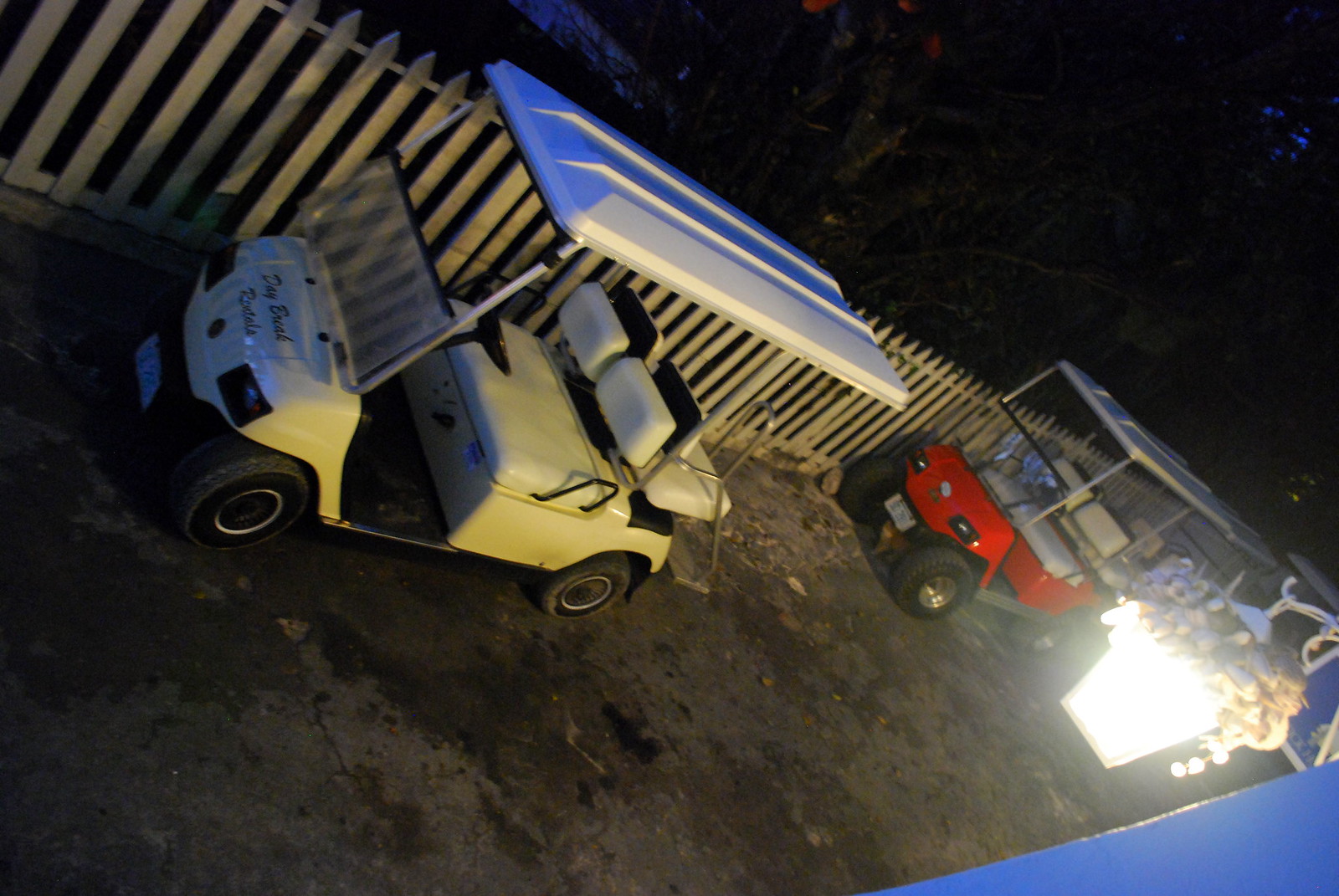The outdoor night-time image is captured at a skewed angle, giving a tilted appearance as if taken from an elevated vantage point. Dominating the foreground, there are two golf carts parked on a dirt surface in front of an off-white picket fence. The golf cart closest to the camera is white with white seats and a white plastic top, marked with "Daybreak Rentals." Directly behind it is a red golf cart, also featuring white seats and a white top, and it appears longer, possibly seating up to eight people. The scene is illuminated by a large, bright white light, emanating from a blue building on the right side. This light is housed in a white metal sconce adorned with shell decorations, enhancing the beach town vibe suggested by the lighting. The backdrop beyond the fence is pitch black, with the faint suggestion of trees.